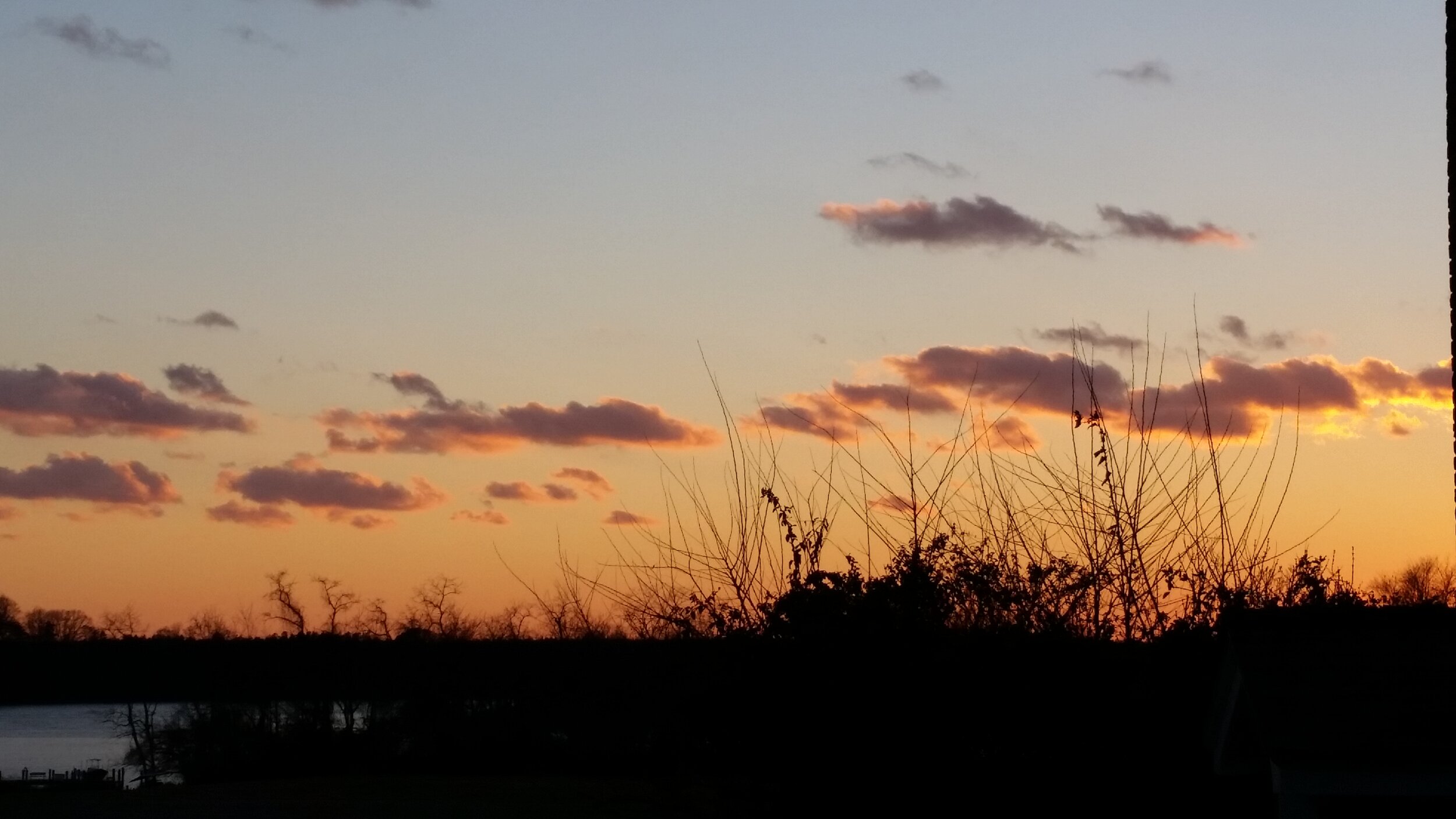This horizontal, rectangular landscape photograph captures the serene beauty of an outdoor scene at sunset. The sky, transitioning from soft blue to a vivid mix of orange and yellow at the horizon, is filled with clouds that range from puffy lavender to gray, reflecting the warm hues of the setting sun. Silhouetted against this colorful backdrop are bare, leafless tree trunks, suggesting a fall or winter season. In the foreground, darkened plant life—consisting of tall grasses, spiky weeds, and twigs—creates a sharp silhouette that adds depth to the image. Beyond the field of blackened vegetation, a body of water glimmers in the distance, its specifics unclear but adding a tranquil element to the scene. The overall color palette is dominated by the deep contrast of orange and black, perfectly capturing the peaceful transition from day to night.